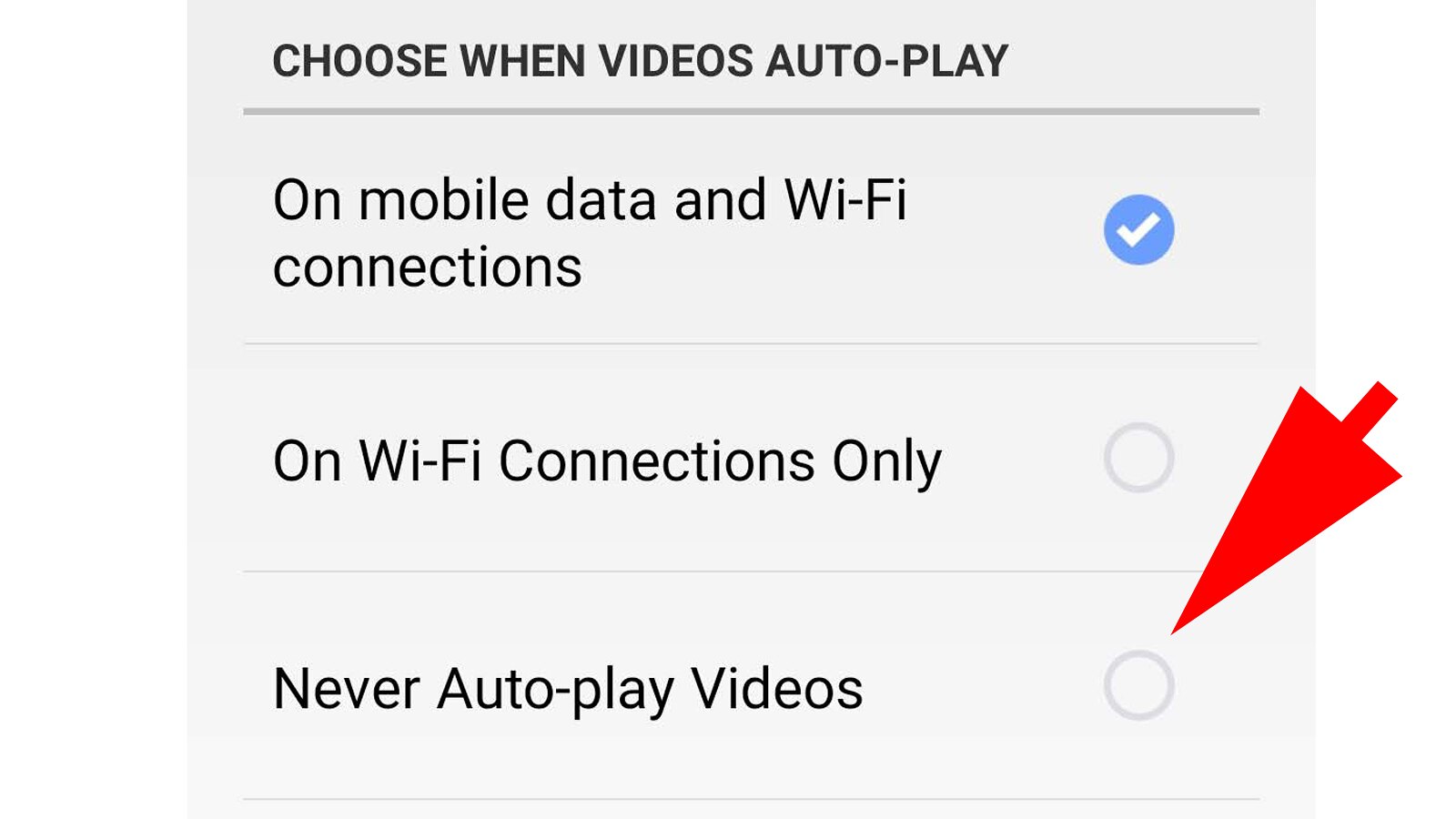A screen capture displays a choice box from a device, either a cell phone or computer. The choice box has a gray background and presents three options. At the top, in black all-capital letters, it reads, "CHOOSE WHEN VIDEOS AUTOPLAY." Below this, a gray line separates the title from the options. The first option, in black mixed case lettering, states "On mobile data and Wi-Fi connections." This option is accompanied by a circle that is checked and highlighted blue. The second option, also in black mixed case lettering, reads "On Wi-Fi connections only." This option features a gray circle that is unchecked. The final option, "Never autoplay videos," is in black mixed case lettering and features an unchecked gray circle. A large red arrow points directly at this last option's circle, suggesting that the viewer should select "Never autoplay videos" and uncheck "On mobile data and Wi-Fi connections."